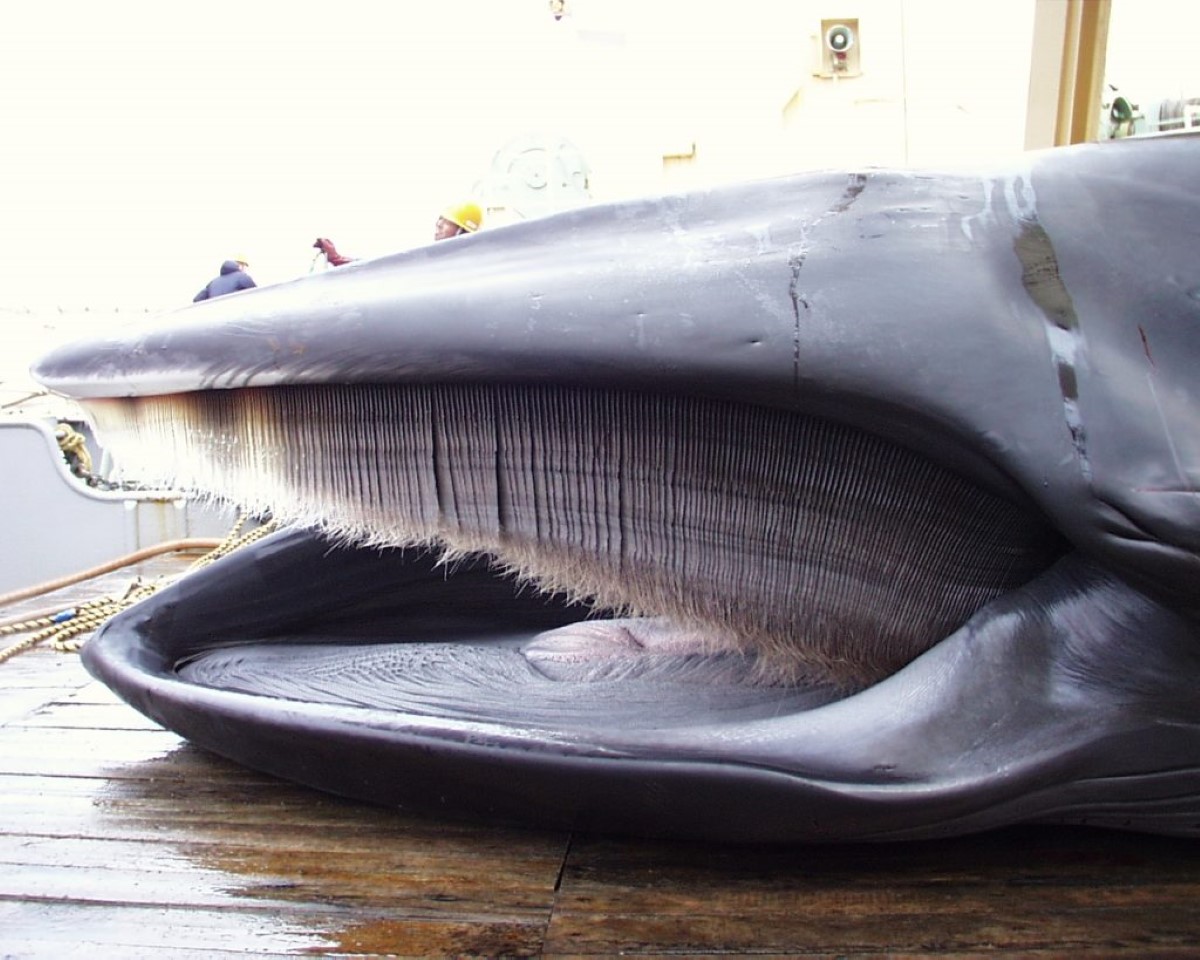This high-definition, zoomed-in photograph captures the head of a gray baleen whale lying on a wet, brown wooden dock, likely a fishing or whaling dock. The whale's mouth is open, prominently displaying its baleen filters hanging from the top jaw, and its tongue and lower jaw are clearly visible. The detailed image reveals the textured pot marks on the whale's skin. Behind the whale's mouth, men wearing yellow hard hats and gloves can be seen, with one also in a dark hooded raincoat, suggesting they might be workers or fishermen involved in handling the whale. To the left, yellow ropes and a gray metal boat, likely a fishing or whaling vessel, are visible. The upper part of the image is slightly blurred, showing what appears to be a loudspeaker and parts of a ship, enhancing the scene's maritime context.